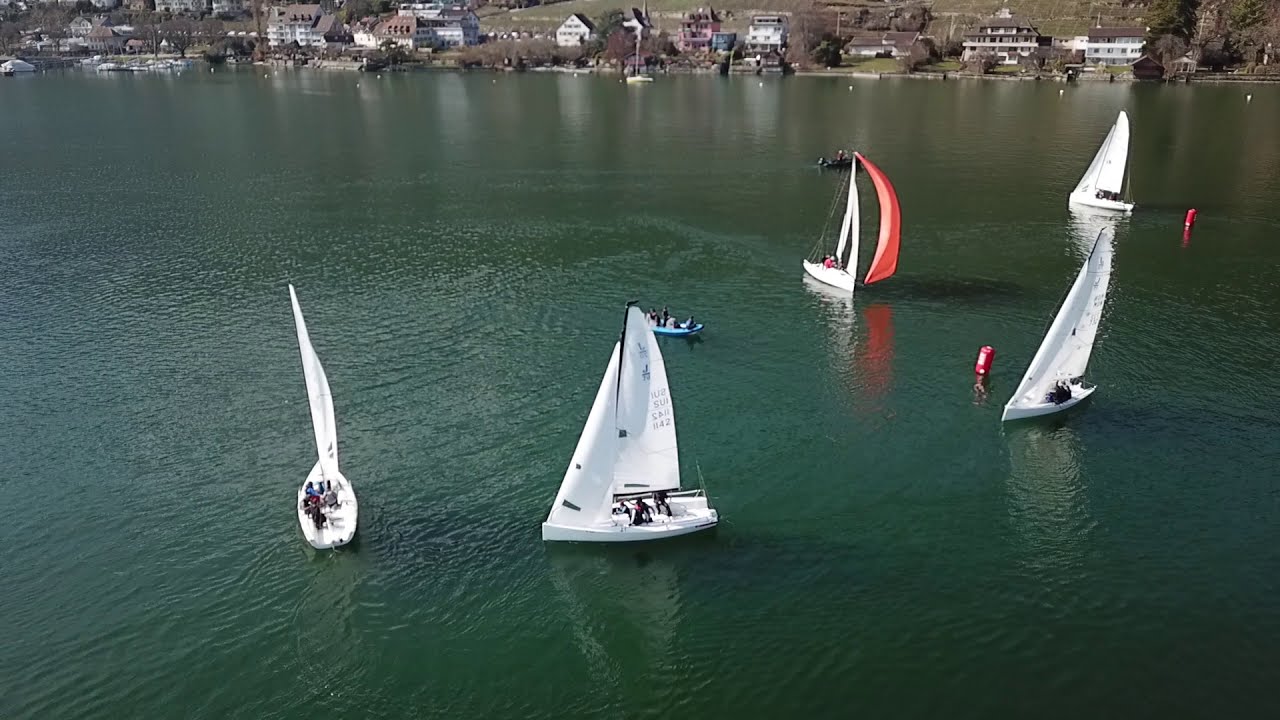In this picturesque scene, a serene lake with dark green, calm waters spans across the foreground, dotted with five distinct sailboats and several smaller vessels. Four sailboats, their white sails catching a gentle breeze, are joined by a striking one boasting a red sail and mast, creating a vivid contrast. These boats appear to be engaged in a leisurely sail, possibly maneuvering around red buoys dispersed in the middle and right sides of the image. Interspersed among the sailboats are two smaller boats, one of which looks like a kayak, and another, perhaps a motorboat, floats in the background.

The shoreline stretching along the top of the photograph reveals a quaint, old town with an array of houses and structures, possibly including a restaurant suggested by the docked boats, exuding an inviting charm. The verdant landscape suggests an autumn setting, with subtle hints of brown foliage peeking through, enhancing the town's tranquil ambiance. The seamless blend of water, boats, and the historical town creates a serene and timeless visual narrative.